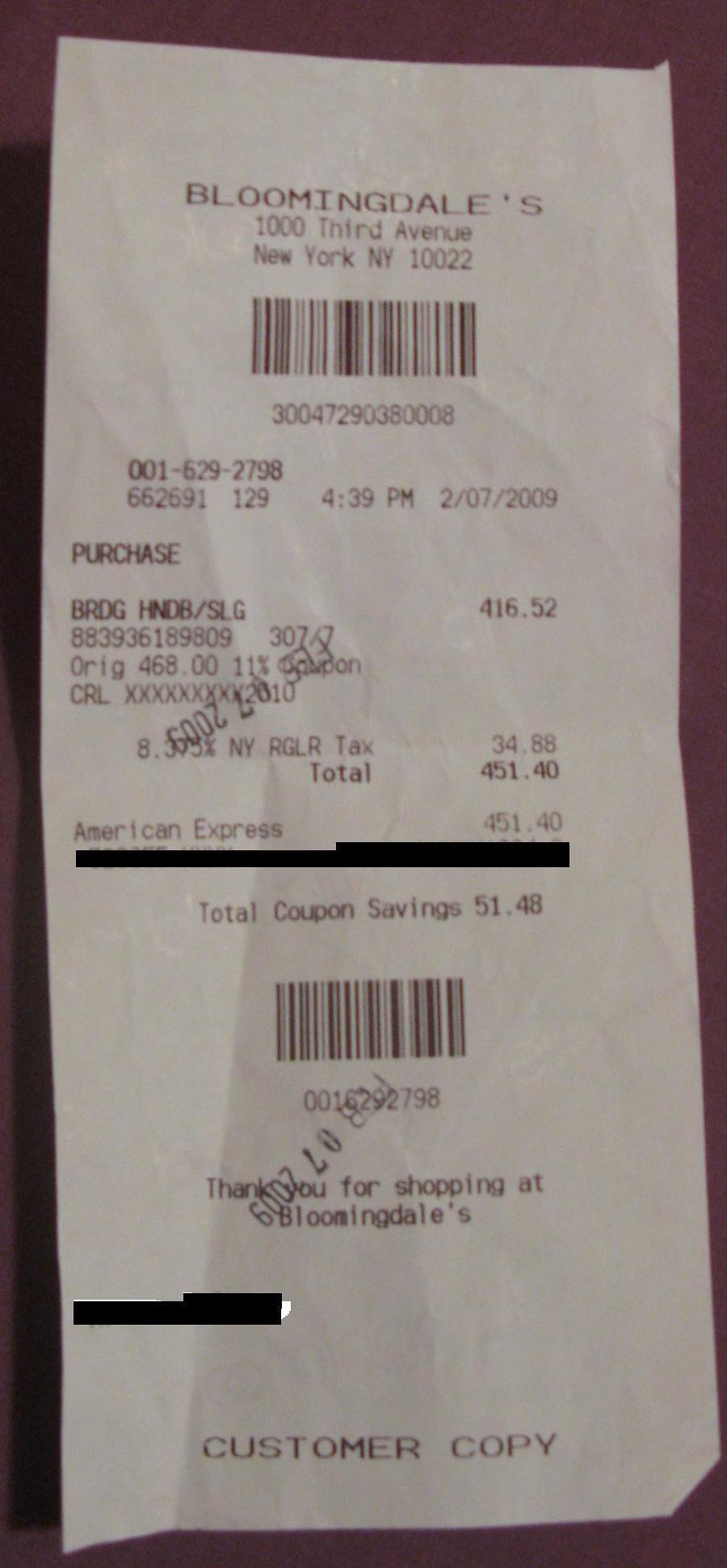This photograph showcases a long, white receipt from a shopping trip at a retail store, resting against a dark maroon background. At the top of the receipt, the store's information is prominently displayed: "Bloomingdale's, 1000 3rd Avenue, New York, New York, 10022." Just below this, a barcode is visible along with purchase details and a SKU number. The receipt indicates that a handbag was purchased for $416.52, with additional tax bringing the total to $451.40. The shopper benefited from a coupon, saving $51.48 on their purchase. Certain personal details, such as the credit card number, have been blocked out for privacy.